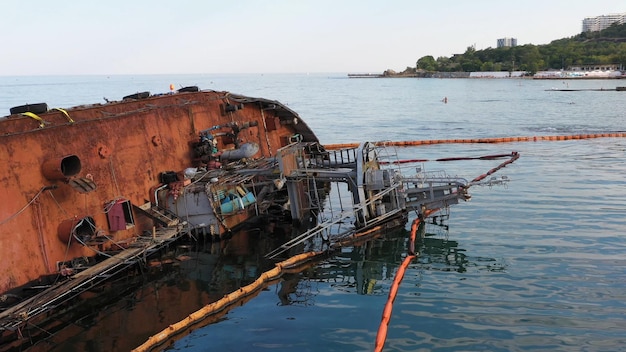The image captures a landscape of a seemingly abandoned and heavily rusted old ship, turned over on its right side and partially submerged in a shallow, coastal body of water. The ship's hull, which is a deep rusted orange color, leans to the left, while various metal pieces, including the mast and towers, jut out and tilt rightward above the waterline. In the foreground, a line of buoys stretches across the image, acting as barriers or markers around the ship, with more buoys visible further beneath the water, extending towards the viewer. The backdrop reveals a vibrant mix of nature and urban development; a verdant peninsula adorned with trees, bushes, and other plant life gives way to modern buildings, likely office structures, and culminates in the impressive silhouette of several skyscrapers against the horizon.